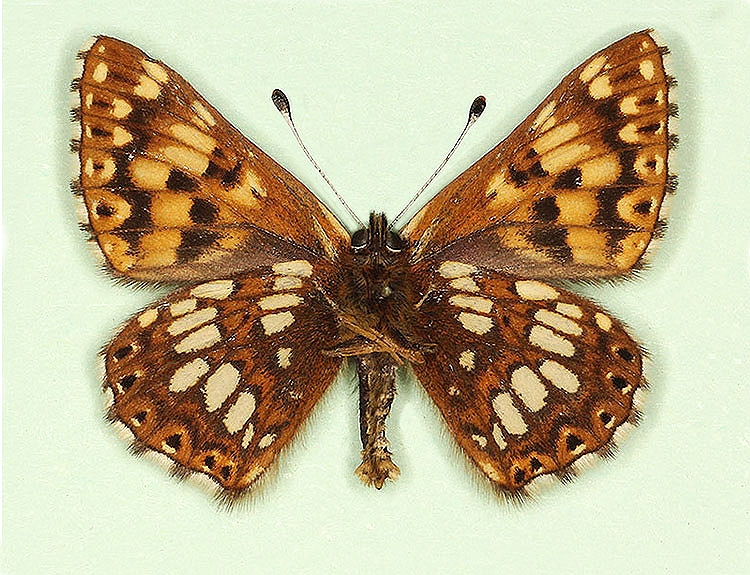The image depicts a seemingly deceased moth laying flat against a light green surface, casting shadows just below its four outstretched wings. The moth is marked by a long, thin, hairy brown body, with legs faintly visible crossed over its midsection. On its head, two antennae jut out at approximately 45-degree angles, black at the tips transitioning into a lighter color. The moth is adorned with a complex mottled pattern on its wings, a mix of brown, orange, black, cream, yellow, and tan colors. The upper wings are primarily reddish-brown adorned with white and black spots, while the lower wings are darker with larger white and tan spots interspersed with bits of black. The detailed and intricate coloration makes for a visually striking display against the light green background.